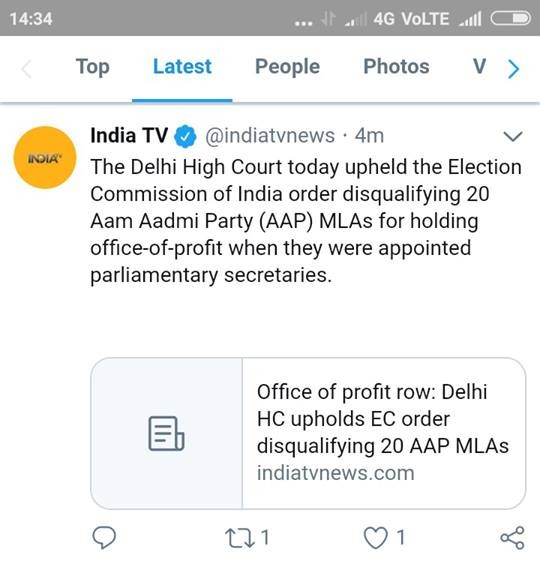This image is a screenshot taken from a cell phone, showing several details at the top, including the device's 24-hour time set at 14:34. The signal strength indicator shows 2 bars, and the device is connected to a 4G network. Another set of bars signifies a full Wi-Fi signal. At the top, there's a heading labeled "Top Latest People Photos in V," suggesting various categories to choose from, with "Latest" visibly highlighted in blue, indicating it is currently selected.

The central focus of the screenshot is a post from an account named "India TV," accompanied by the hashtag #IndiaTVNews. The account's avatar is yellow, featuring the word "INDIA" in a black gradient. The post was published 4 minutes ago and is styled as a tweet, possibly from a platform like Twitter or Meta. The content of the post reads: "The Delhi High Court upheld the Election Commission of India order disqualifying 20 Aam Aadmi Party (AAP) MLAs for holding office of profit when they were appointed Parliamentary Secretaries." Additionally, there is an attached document titled "Office of Profit Row: Delhi HC Upholds EC Order," allowing users to open and read more details. The post also shows minimal engagement, having been shared and liked only once.